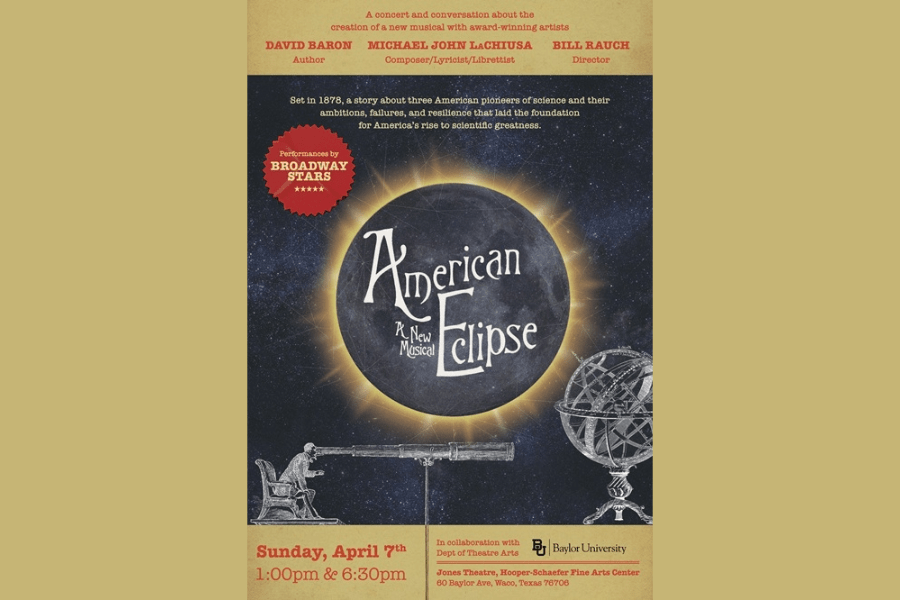This is a detailed Broadway poster for the musical "American Eclipse," featuring a dramatic image of a large eclipse with the sun shining behind the moon in the center. The background is gold with a superimposed black rectangle. At the top of the poster, red text announces "A Concert and Conversation about the Creation of a New Musical with Award-Winning Artists." The artists named are David Baron (author), Michael John LaChiusa (composer and lyricist), and Bill Rauch (director). Above the eclipse is a red circle stating "Performances by Broadway Stars." The lower part of the poster includes a scene of a man sitting in a chair, gazing through a telescope at a steel globe to his right, symbolizing the trajectory of celestial objects. Event details at the bottom of the poster specify the date and time: Sunday, April 7th, at 1 p.m. and 6:30 p.m. The venue is listed as Jones Theatre, Hooper Schaeffer Fine Arts Center at Baylor University, Waco, Texas.